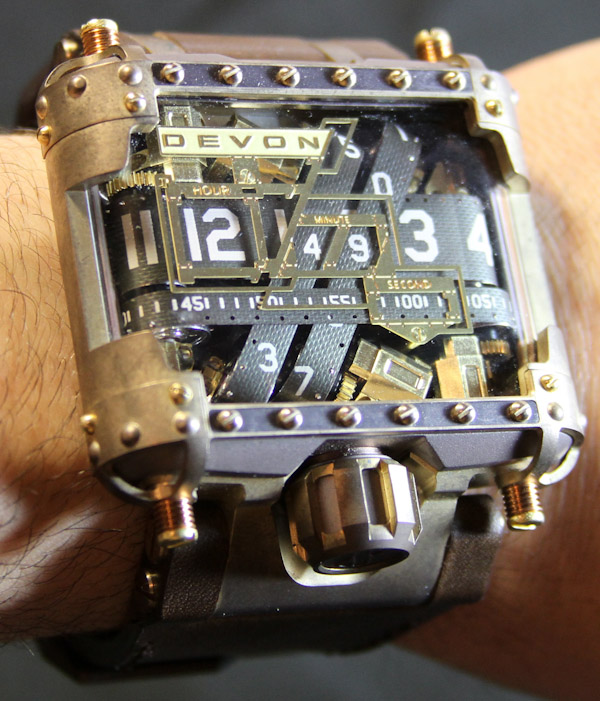The image depicts a distinctive and intricate Devon branded watch, prominently displayed on a man's wrist against a black background. The watch has a mechanical, steampunk aesthetic, characterized by visible bolts and screws along its edges. Housed in a square metallic casing, the timepiece displays the current time as 12:49:34, with the seconds counting visibly on a belt system. The design showcases various numbers and gears that highlight its complex inner workings as they change with the time. The watch features a black band, adding to its industrial and hardware-rich appearance. The detailed metallic construction, combined with the exposed mechanical elements, creates a visually striking piece that blends functionality with an artisanal, almost futuristic style.